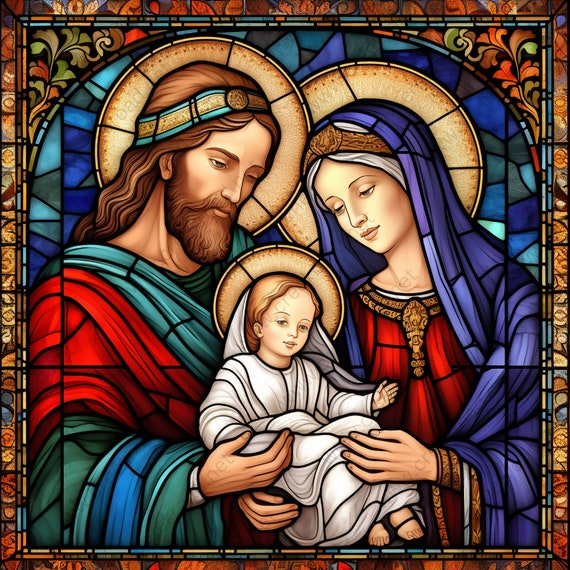This image depicts a digitally created stained glass window, rich in vibrant colors typically associated with religious art. At the center are three figures, likely representing Joseph, Mary, and baby Jesus. The man on the left, clad in red robes with teal and gold details, has long brown hair, a thick beard, and a teal and gold headband. He gazes downward contemplatively. The woman on the right, presumed to be Mary, wears a red dress adorned with ornate gold detailing at the neck and sleeves, along with a long blue cover over her head, also looking down. The baby, possibly Jesus, is dressed in an all-white robe and has light brown hair. Each figure is encircled by halos, enhancing their holy depiction. The background features a blue arch and a variety of leaves, framed by a colorful, detailed border. This meticulously crafted artwork captures the essence of stained glass windows found in churches, emphasizing its sacred and visually striking qualities.